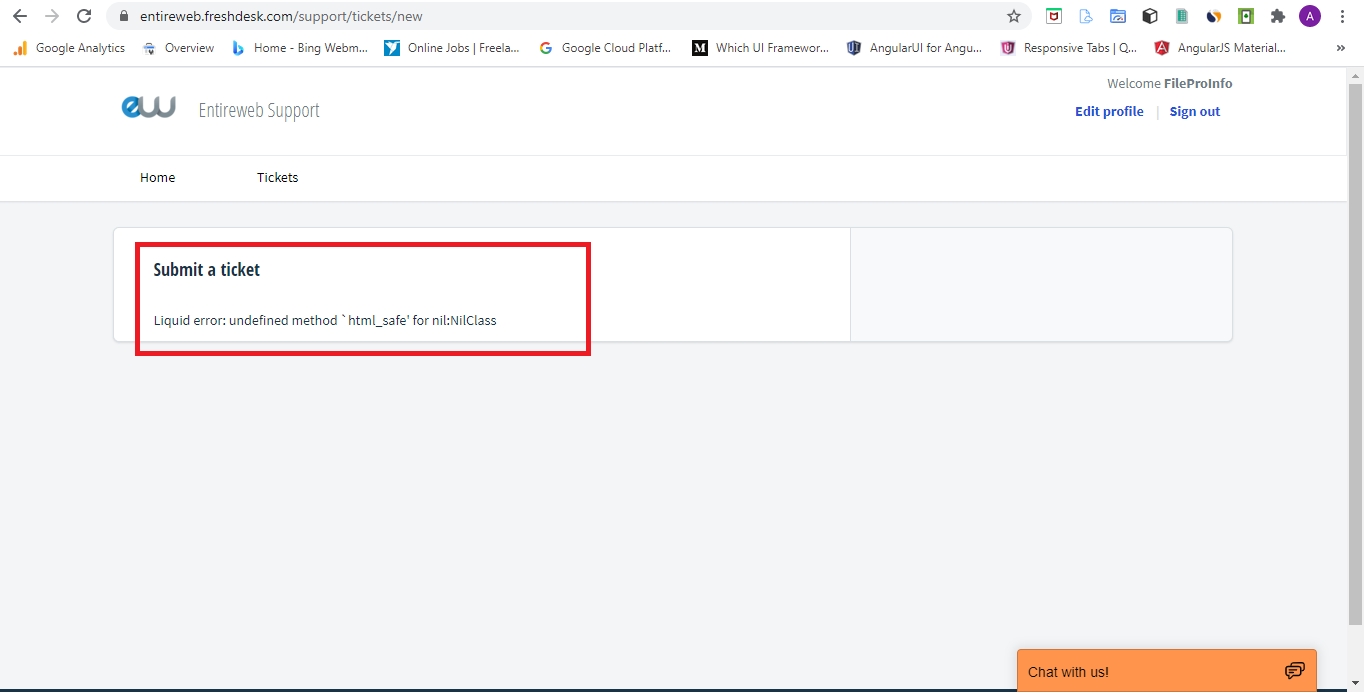The image depicts a screenshot of a computer screen featuring a webpage with an all-white background. The bottom half of the screen has a very light gray shade. At the top of the screen, there are navigational buttons including 'Back,' 'Forward,' and 'Retry.' Additionally, there's a URL bar for entering web addresses, flanked by various icons on the right side in a single row. Below this row, another row contains multiple clickable tabs. 

Centrally located on the page is a large white rectangle displaying a local logo, which consists of a blue "E" followed by a gray "W." To the right of the logo, the text "Entire Web Support" appears. Adjacent to this, there are blue links labeled "Edit Profile" and "Sign Out." Directly beneath, two tabs allow users to choose between 'Home' and 'Tickets.' In the light gray section of the screen, another large white rectangle is labeled "Submitted Ticket," with additional text that reads "Liquid Air" followed by illegible content, all encased within a red rectangle.

In the bottom right corner, an orange rectangle with black text prompts users to "Chat with Us" and features an icon of two conversation bubbles. A scrollbar is visible on the right side of the screen, indicating that the page can be scrolled vertically.